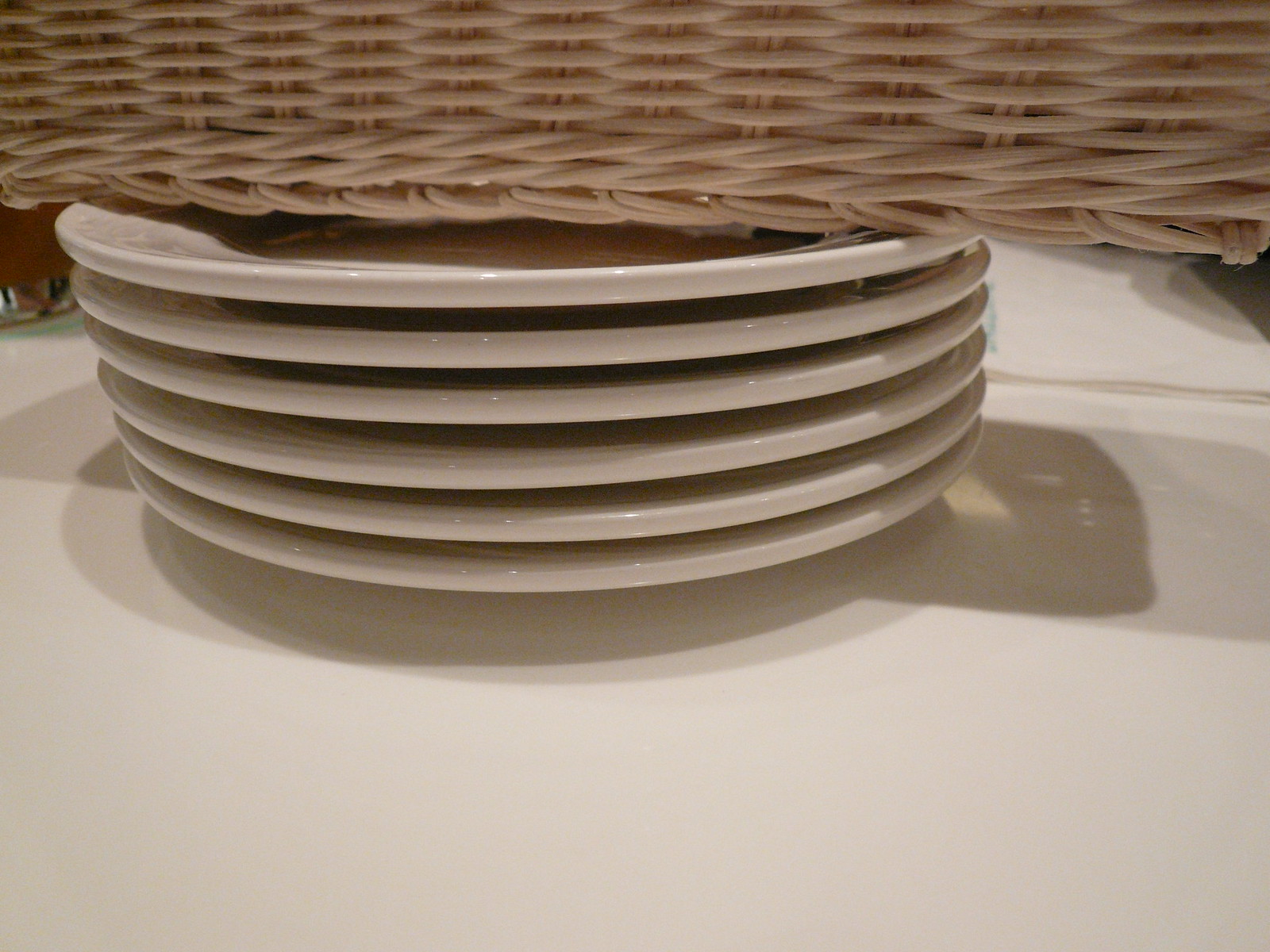In the image, there is a pristine white table illuminated by light that casts a shadow. At the center of the table, six glistening, white ceramic plates are neatly stacked. Resting atop this stack, almost as if it's utilizing the plates as a stand, is a light tan, newly manufactured wicker basket. The basket's woven texture and meticulous construction suggest it is unused, much like the plates beneath it. To the left near the top, there is a glass containing a brown liquid. The interplay of light and shadow underscores the cleanliness and newness of the items, creating an aesthetically pleasing arrangement.